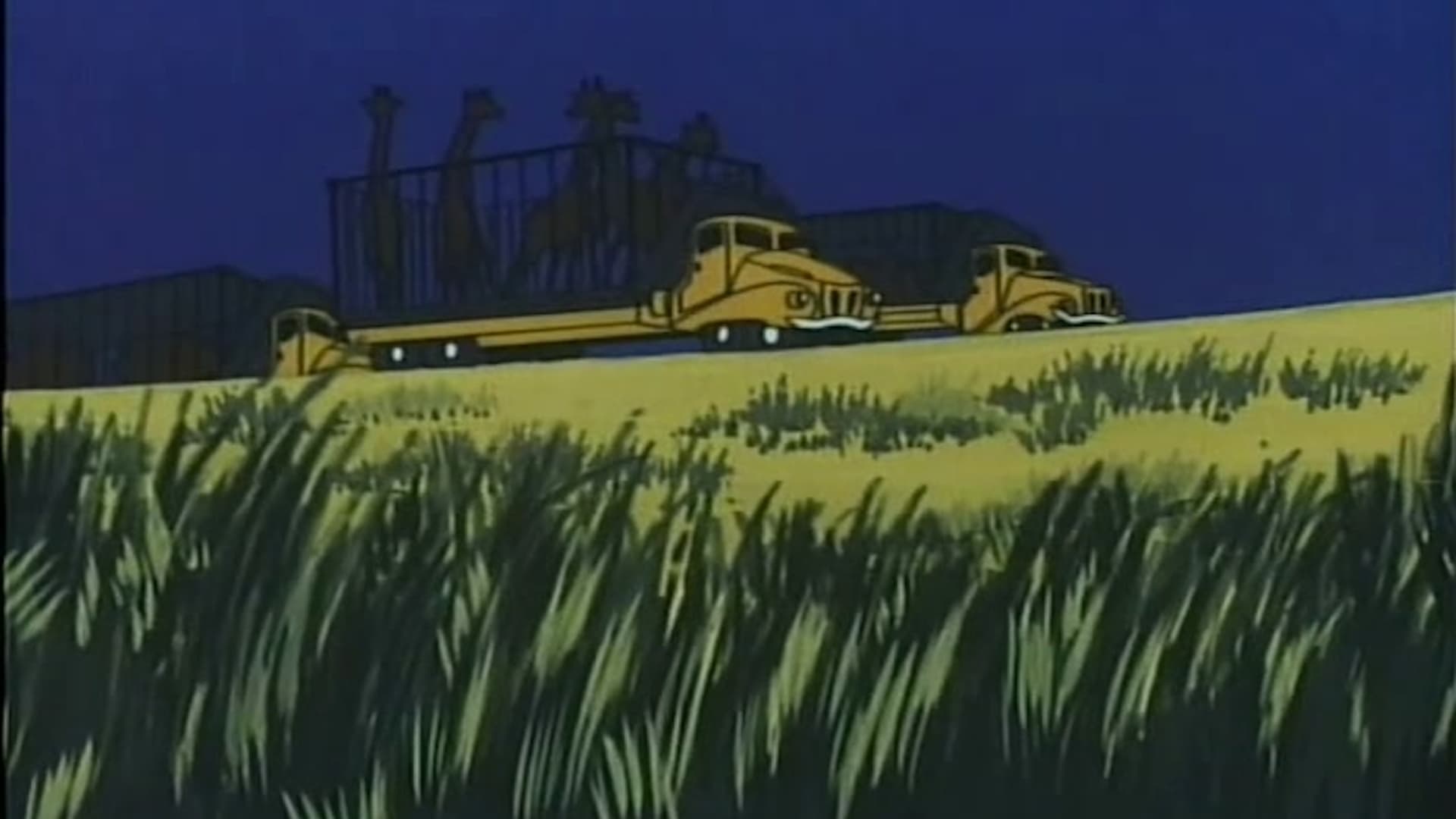This image is a cartoon still from what appears to be an old-style animation, possibly from the 1980s. It depicts a grassy prairie field with no trees in sight. At the top of the grassy area, three large, yellow trucks are driving on a road. The trucks, which have a rounder, older style design with protected wheelbases, are prominently featured. Each truck has a different cargo: the truck in the center foreground carries six giraffes in a steel cage without a roof, allowing the giraffes' necks to extend out. The truck behind it has a metal trailer with two large animals and a roof. The third truck, partially visible on the side, has metal containers on its back. The trucks have a total of four wheels in the front and eight in the back. The sky in the background is a deep, dark blue, providing a stark contrast to the bright yellow trucks and green field below.